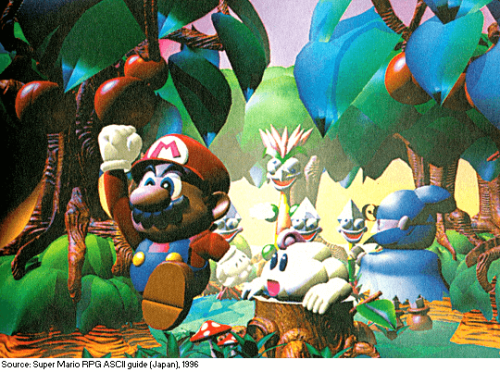The image is a vibrant illustration from the 1996 video game "Super Mario RPG," showcasing a colorful and whimsical forest scene with cartoon characters. Central to the image is Super Mario, easily identifiable by his signature red hat adorned with an "M," a matching red shirt, blue overalls with yellow buttons, and white gloves. Mario is dynamically depicted marching to the left, one leg lifted and a fist raised triumphantly in the air. His iconic mustache and large nose are prominent, adding to his familiar look.

Surrounding Mario are a variety of creatures and elements characteristic of early polygonal 3D design. To his right, perched on a tree stump, is a distinct little white blob with black eyes and a pink mouth, engaging the viewer with its curious gaze. Further in the background, there are more nondescript, puppetry-like creatures in yellowish-beige hues, adding to the fantastical environment. The scene is lush with trees bearing green leaves and vibrant red fruits that resemble apples, contributing to the dense and lively forest setting.

The ground beneath Mario's feet is depicted in a unique yellow tone, complementing the overall bright and abstract style of the artwork. The image is framed by text at the bottom-left corner, which reads: "Source: Super Mario RPG ASCII Guide, Japan (1996)." This caption not only anchors the artwork in its video game origins but also lends a nostalgic touch to the vividly rendered scene.